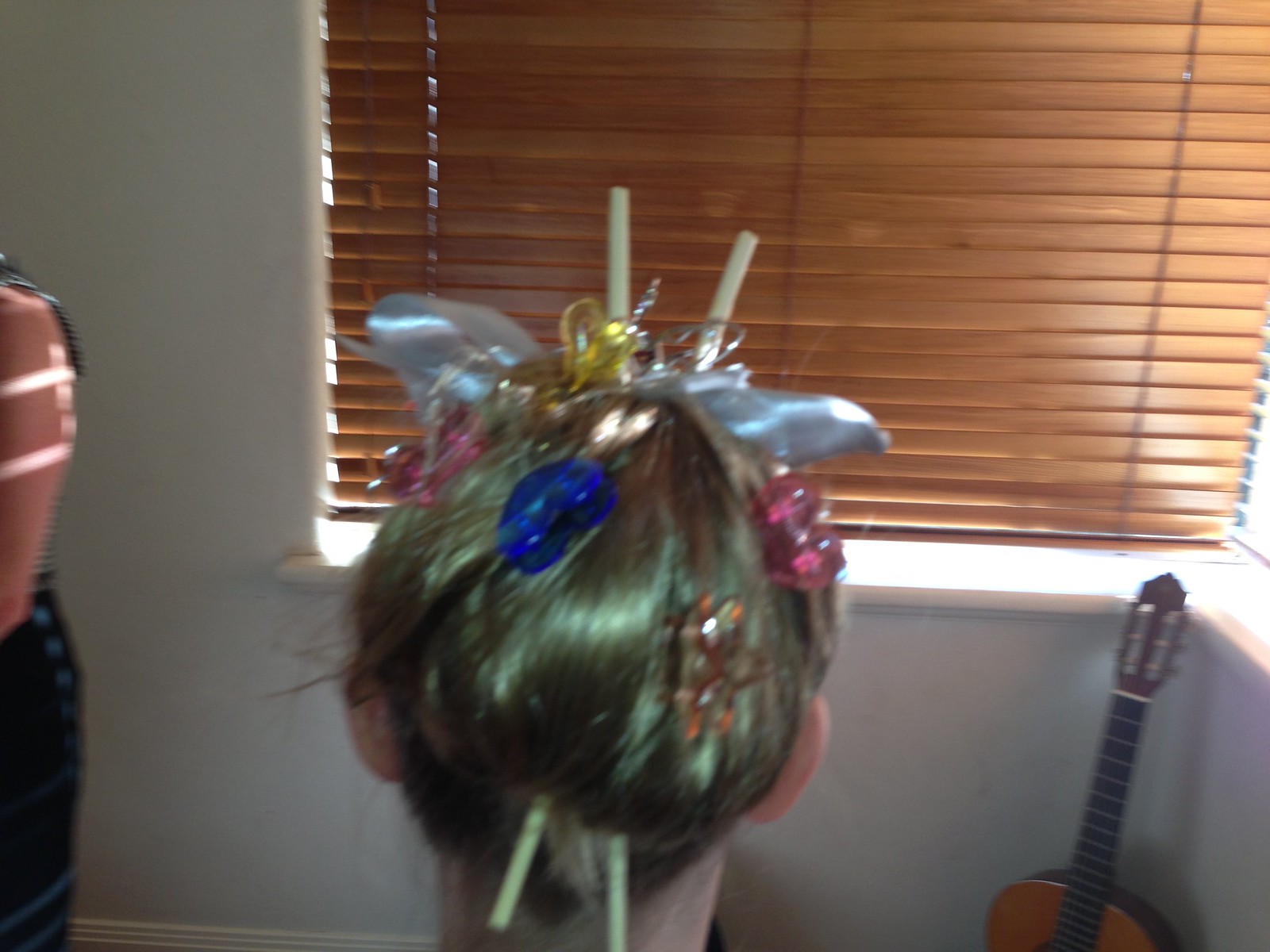A somewhat blurry indoor photograph captures the back of a young person's head, possibly a girl or teenager, with blonde hair styled in a bun. The hair is adorned with colorful plastic barrettes—pink, orange, blue, and even a yellow one—and a shiny metallic silver headband. Additionally, two long sticks, resembling lollipop sticks or thin sewing needles without tips, are arranged in an X shape through her hair. The scene also includes a brown window with golden blinds that are drawn, allowing a slight peep of sunlight through. Partially visible is an acoustic guitar propped up against the corner of a counter on the right side, adding a touch of coziness to the simple indoor setting with its plain white walls.